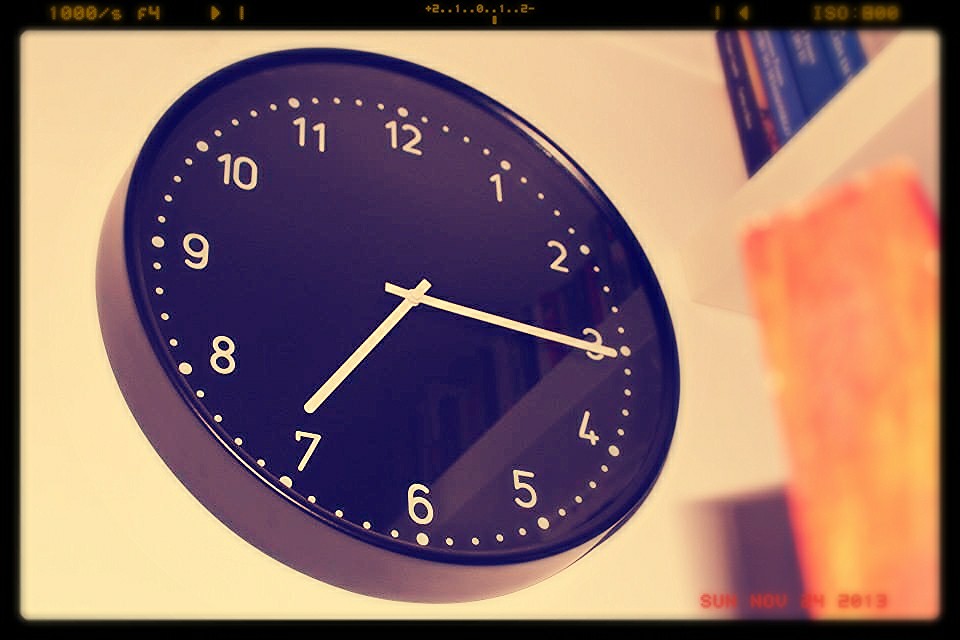This color image features a close-up of a light brown-housed clock mounted on a light pink wall. The clock face is black with large white numbers and a combination of big white circles next to the numbers and smaller circles for the minute markers. The hour hand is slightly past the 7 while the minute hand is at the 3, indicating the time is 7:15. The photograph also captures, in the lower right-hand corner, a timestamp in red text that reads "Sunday, November 24, 2013." To the right of the clock, there is a white bookcase with several books, including dark blue and cyan blue ones with white lettering, and a large piece of light brown wood.